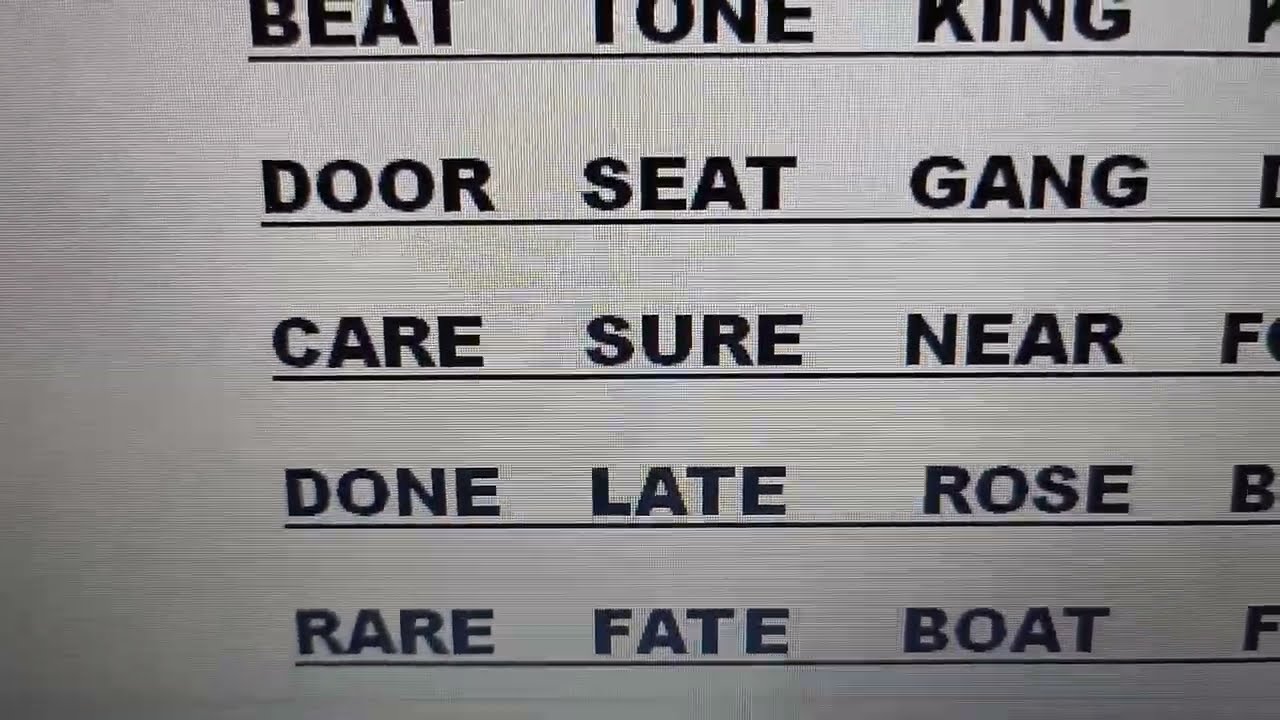The image depicts a white background on a computer screen, captured photographically rather than as a direct screenshot, displaying five rows of bold, black, uppercase four-letter words. Each row consists of three fully visible words followed by a partially visible fourth word. The words are not in alphabetical order and do not seem to carry specific definitions or contextual hints. The first row reads "BEAT, TONE, KING," the second row "DOOR, SEAT, GANG," the third row "CARE, SURE, NEAR," the fourth row "DONE, LATE, ROSE," and the fifth and final row "RARE, FATE, BOAT." The font appears to be Times Roman, and some horizontal lines are visible across the image due to the photograph of the screen. There are beginnings of additional words on the far right of each row, but only their initial letters (such as 'F' or 'B') are visible. No people or other elements are present in the background.